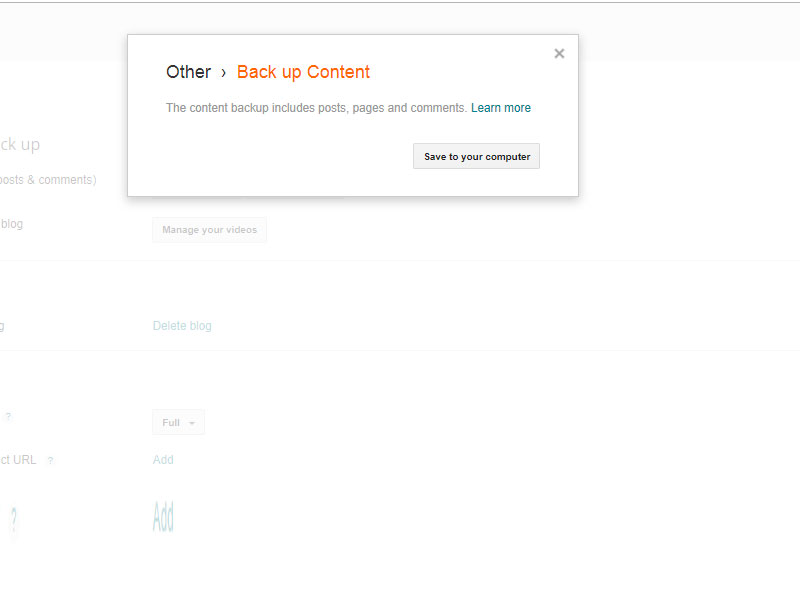The image depicts a computer screen showcasing a webpage with a prominent pop-up notification at the center. The pop-up message highlights "Other Backup Content" and specifies that the content backup includes posts, pages, and comments. Below this information, there's an option labeled "Learn More" followed by a button labeled "Save to Your Computer." The background of the screen features the CK app interface, which displays various details that appear blurry as the focus is on the pop-up message in the foreground. The repeated "Learn More" signs emphasize the availability of further information.